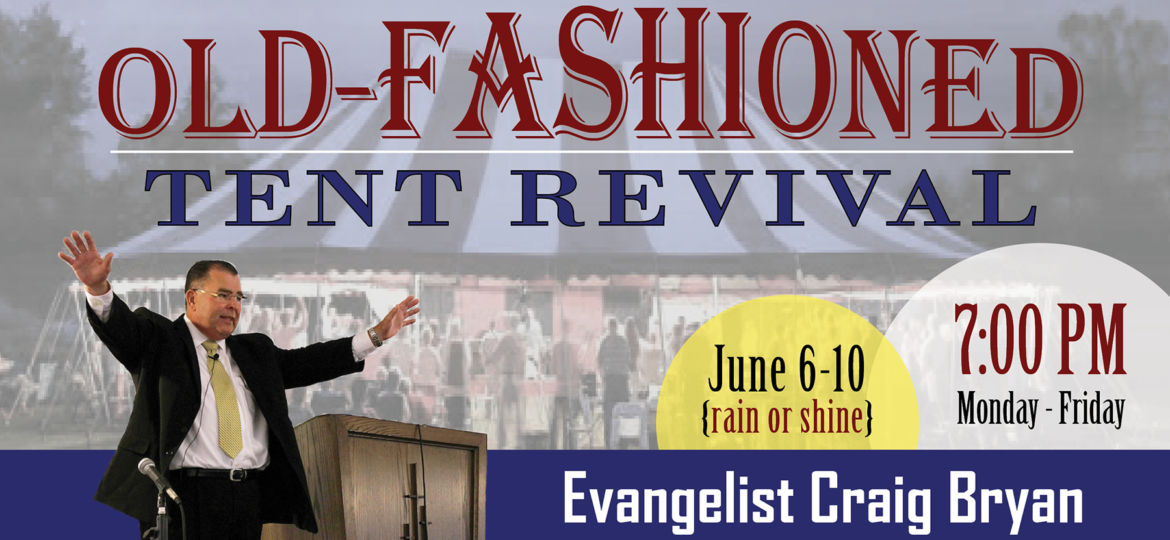The advertisement prominently features the heading "Old Fashioned Tent Revival" with "Old Fashioned" in red and "Tent Revival" in blue. The background image depicts a large tent filled with people, suggesting a lively religious gathering. In the bottom left corner, there is a white-skinned man, possibly in his 50s, identified as Evangelist Craig Bryan. He is dressed in a black suit with a white button-down shirt and a yellow tie, glasses, and has a microphone attached to his tie. He stands with his arms outstretched near a wooden podium. In the bottom right corner, event details are provided in white text, mentioning the dates June 6th through 10th, rain or shine, at 7 p.m. Monday through Friday. The information is accentuated with yellow circles and a horizontal red stripe highlighting the evangelist's name and the event schedule.